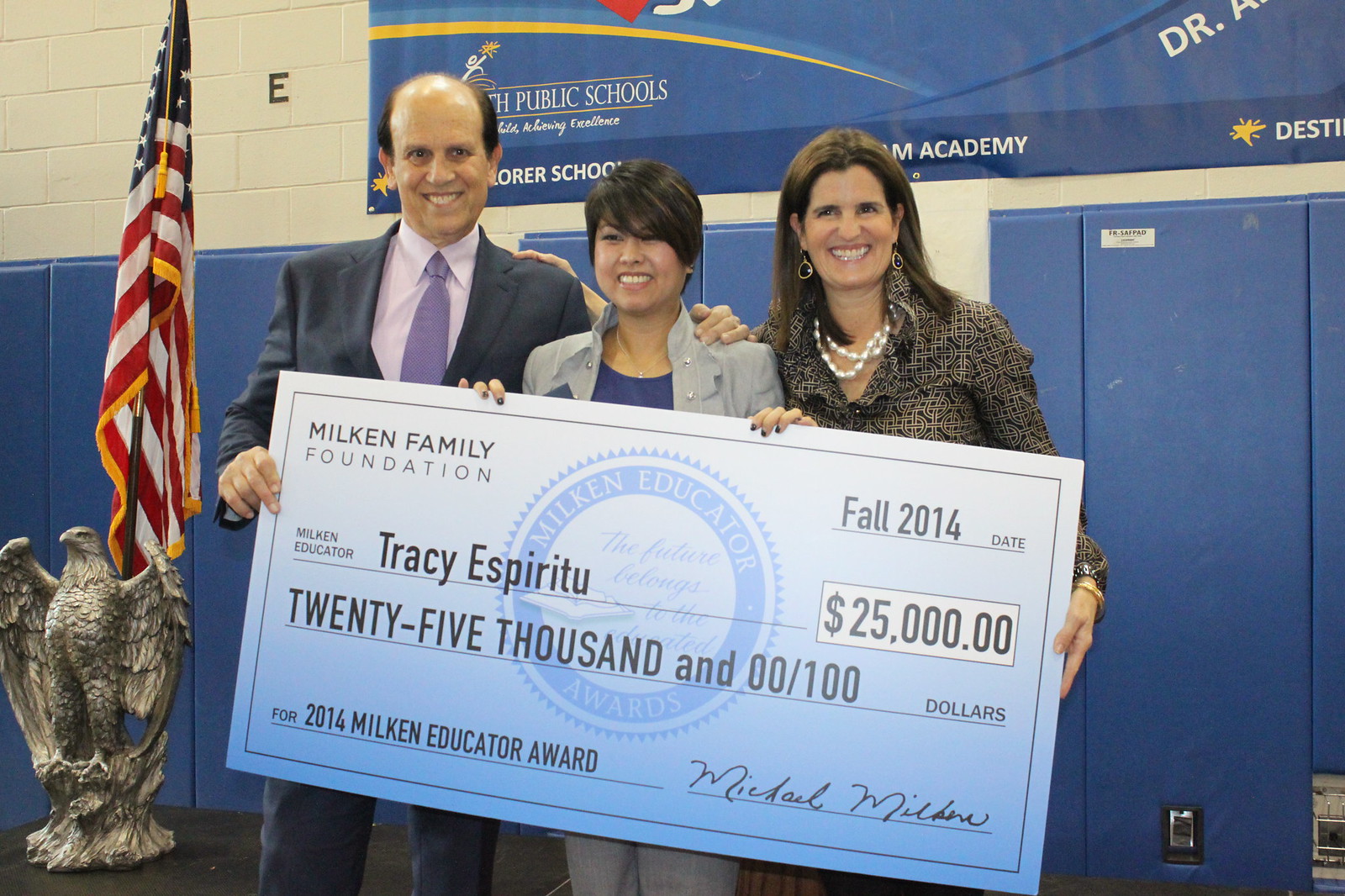In this horizontally aligned rectangular photograph, three adults stand in what appears to be a gymnasium, evidenced by the presence of blue mats on the walls, blue lockers, and a white brick wall above, partially obscured by a blue banner with the words "public schools" and "Academy." The trio is holding a large ceremonial check from the Milken Family Foundation, awarded to Tracy Espiritu, who is likely the woman in the middle. The check, signed by Michael Milken, awards Espiritu $25,000 for the 2014 Milken Educator Award, noted with "Fall 2014" in the upper corners.

On the left, a man with a smile, a bald head, and short black hair on the sides, is dressed in a dark gray suit, white shirt, and a purple tie. Next to him, Tracy Espiritu is also smiling, with short-styled brown hair, a purple collared shirt, and gray pants, holding the check with both hands. To her right, another smiling woman with long straight brown hair, parted in the middle, wears large beaded white earrings, a matching necklace, and a patterned gold and black blouse. Next to the man, there’s a bald eagle statue holding an American flagpole, further indicating the patriotic setting of the photograph.